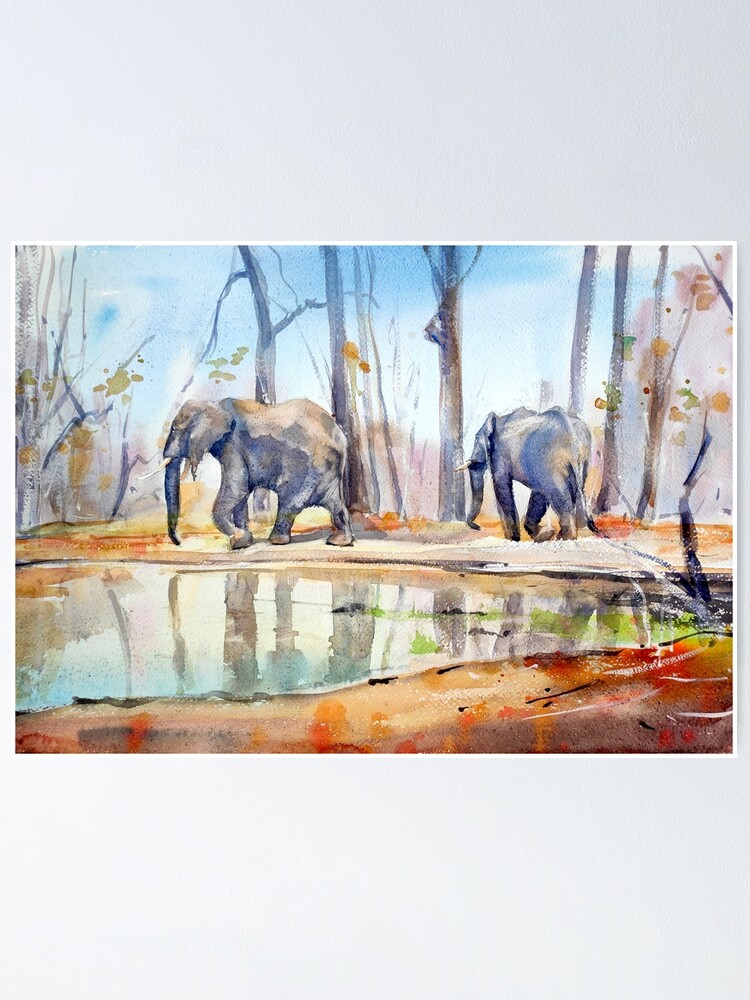The painting depicts a tranquil woodland scene, intricately detailed in watercolor. In the foreground, a shallow pool of water with green shapes and what seems to be wood along the right side reflects the surrounding trees and partially the two gray elephants. The elephants, characterized by their large tusks and trunks, are positioned on the far bank of the pond. The larger elephant on the left walks towards the left side of the image, while the smaller one on the right appears to be moving away from the viewer. The woodland area features tree trunks and sparse foliage, some in fall colors, with a ground that is whitish beige marked with splotches of rust color suggesting fallen leaves. Despite the natural habitat typically associated with grassy plains, this scene intriguingly places the elephants in a forested area. The painting offers a unique juxtaposition of the elephants' typical environment with a woodland setting, enhancing its serene and somewhat unorthodox beauty.